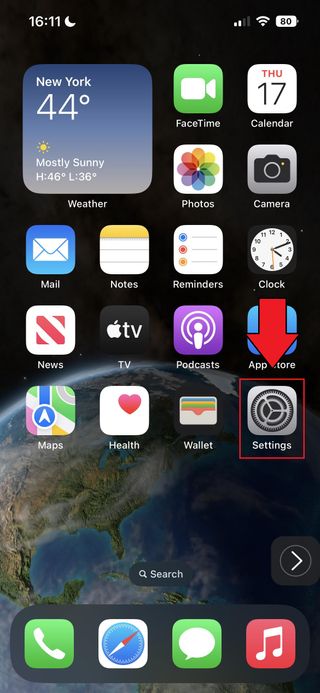A detailed screenshot of a cell phone display at 16:11, indicated by a white time and crescent moon against a black background. The top bar of the screen includes the WiFi signal strength, cell signal strength, and an 80% battery indicator.

The home screen's background displays an image of Earth, focusing on the United States. At the bottom of the screen, a white search bar with a magnifying glass icon labeled "Search" is visible. To the right of the search bar, there's a square icon with an arrow pointing to the right.

Along the bottom dock, the icons for Phone, Safari, Messages, and Music are present. Above these, the display shows the location as New York and the weather information: 44°F, mostly sunny, with a high of 46°F and a low of 36°F.

The screen also features a grid of app icons, including FaceTime, Calendar, Photos, Camera, Mail, Notes, Reminders, Clock, News, TV, Podcasts, and the App Store. Notably, a red arrow pointing down appears over the App Store icon, indicating something important. Additional icons for Maps, Health, Wallet, and Settings are also visible, with the Settings icon highlighted by a thin red square.